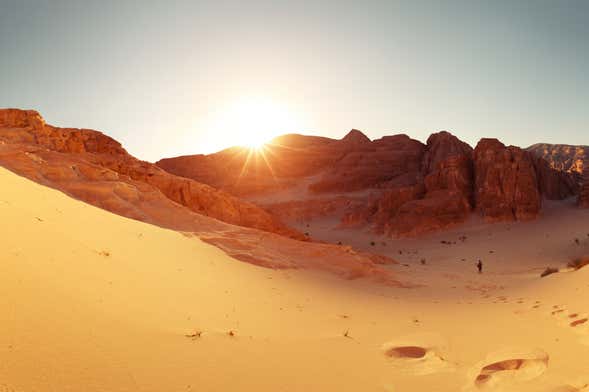This is a photograph of a vast desert landscape at sunset. The bottom half of the image showcases undulating, yellow-golden sand dunes that slope from the top left down to the bottom right. The sand is marked with footprints that extend across the scene, suggesting recent passage. In the middle distance, a couple of tiny, indistinct figures—possibly people—are seen walking on the sand, reinforcing the sense of scale and isolation. The background features rocky formations with a reddish-orange hue, their surfaces marked by cracks and crevices, as well as a striking, darker black rock to the right. The setting sun peeks over these rocks, casting dramatic, elongated shadows and illuminating the landscape with a warm, golden light. The sky above transitions from a pale, greyish-blue to a soft white, devoid of clouds, contributing to the tranquil yet dramatic feel of the scene. The overall composition, captured with a wide-angle lens, emphasizes the sheer expanse and varied textures of this desert environment.